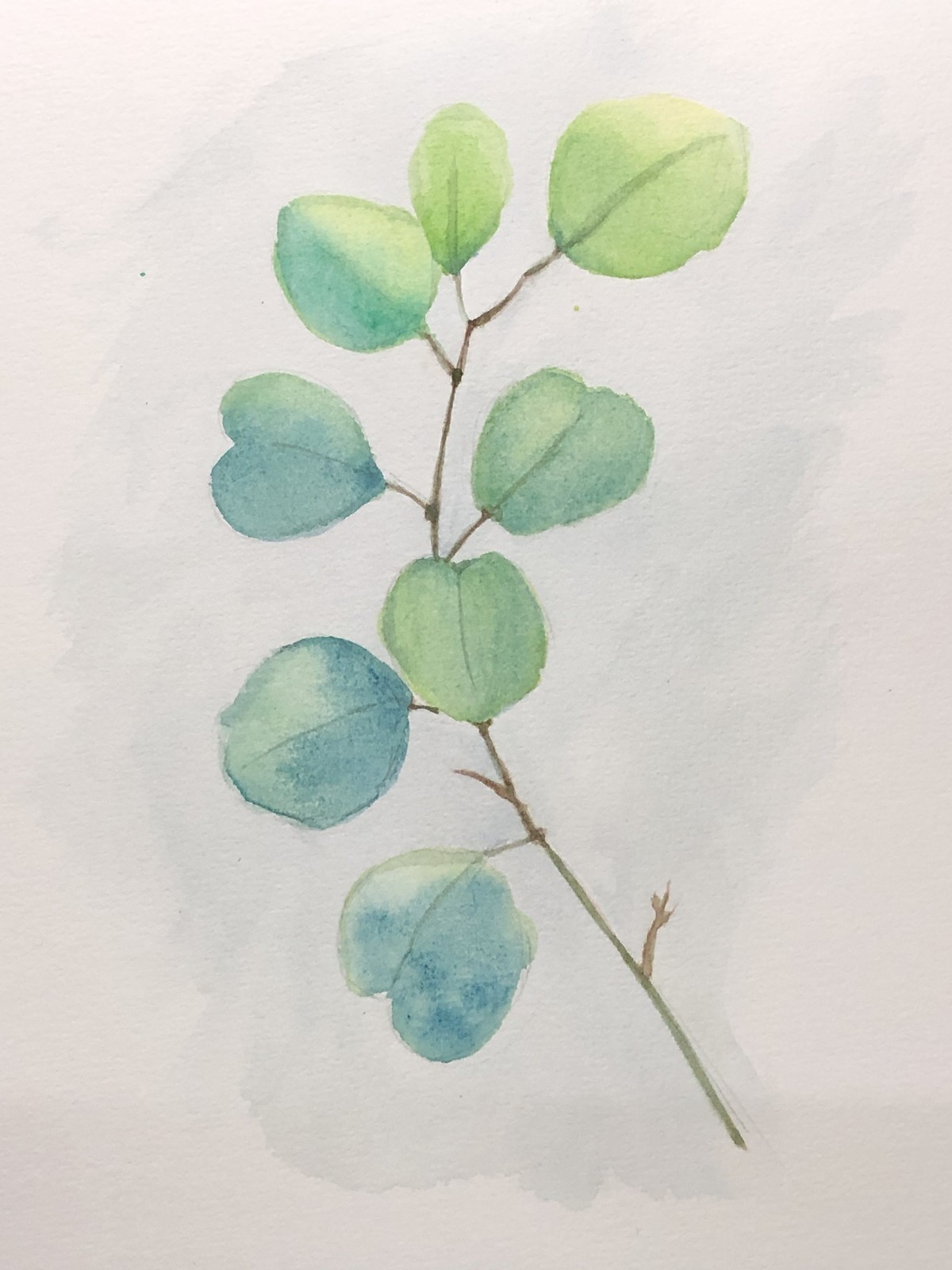The image is a detailed watercolor painting featuring a curved stem or twig ascending from the bottom right to the upper right, adorned with eight leaves in varied tones of green and blue. The background is a subtle blend of white and light blue watercolors, adding depth and a slight shadow effect. The leaves, which range in shape from rounded to slightly heart-shaped, are distributed with five on the left and three on the upper right. The lower leaves exhibit darker blue hues, transitioning to lighter greens towards the top. Each leaf has distinct lines adding dimension, with some showcasing a blend of dark and medium blues alongside the greens, enhancing their flat, pastel-like appearance. The uppermost leaf is particularly notable for its fuller, traditional shape with a defined central vein and a gradient of greens with a hint of blue near its base.